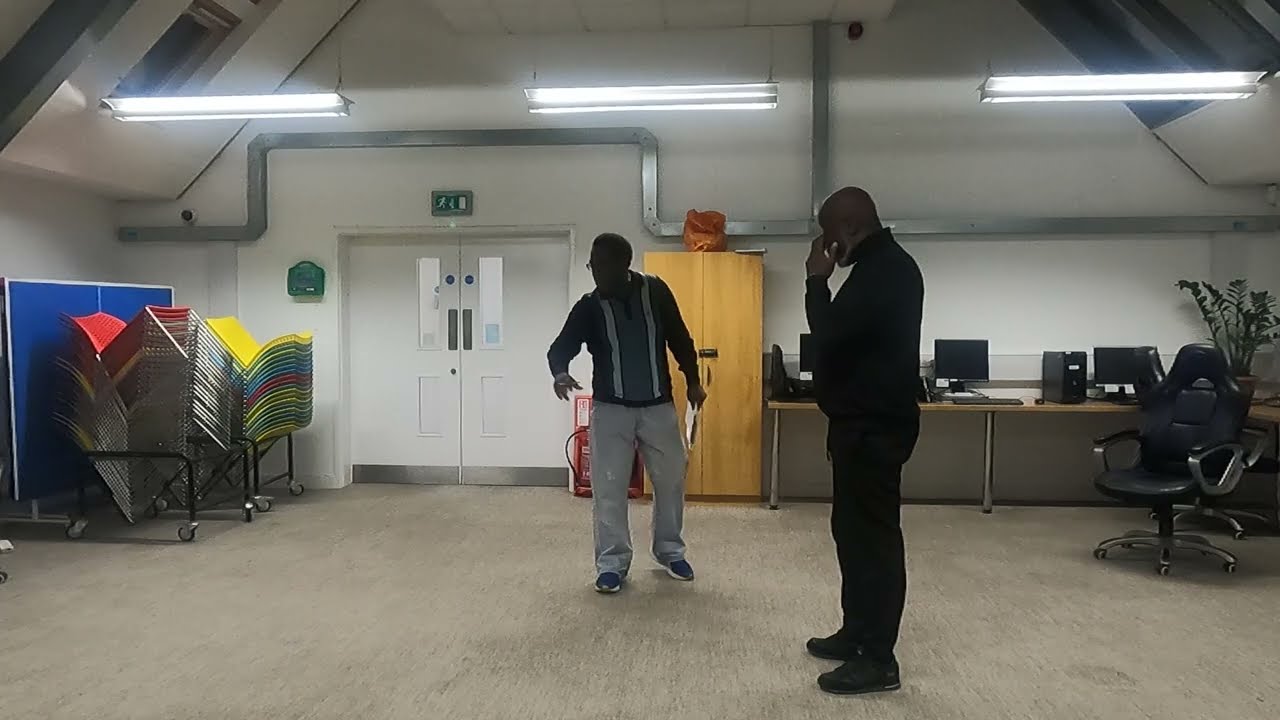The image depicts an interior office space with white walls forming a triangular shape. The flooring appears to be tan, possibly carpet or wood. Centrally located in the room are two men, seemingly engaged in a conversation. The man on the right, attired in black pants, a black jacket, and black shoes, is on the phone. The man on the left, wearing gray jeans with gray shoes that have white bottoms and a long-sleeve gray shirt with light gray stripes, holds a piece of paper while looking to his left.

The back of the room features a desk lined up against the far wall, supported by silver metal legs. This desk houses several black computer workstations. On the right side near the desk, there is a black executive rolling chair, while to the left, there are multiple stackable plastic chairs on rollers. Additional elements in the room include overhead fluorescent lights suspended from the ceiling by wires and a white double door in the background to the left of the image. The scene is lively with colors such as tan, gray, black, red, yellow, blue, green, orange, silver, and white. This setting clearly represents a typical office environment.